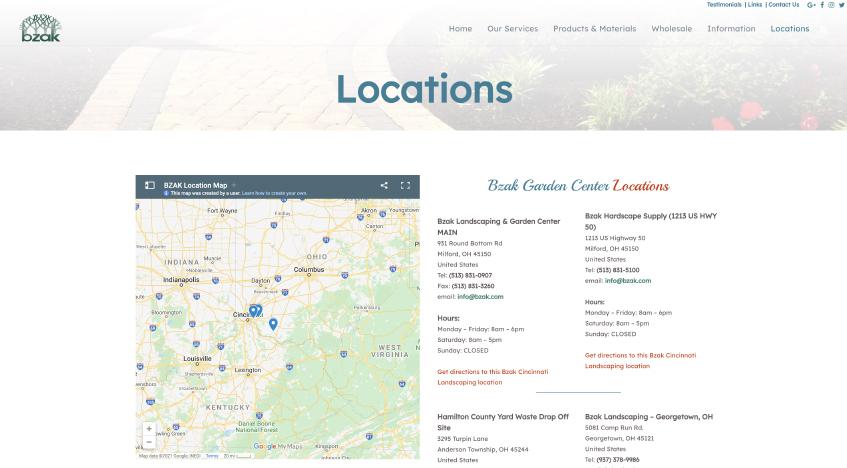The image depicts a webpage from a website called BZAK, with "BZAK" prominently written in the left-hand corner accompanied by small tree icons at the top. The design of the site is simple yet unique. The focal point of the webpage is the bold, centrally placed heading that reads "Locations." 

The navigation menu at the top offers several options: Home, Our Services, Products and Materials, Wholesale Information, Locations (highlighted), Testimonials, Links, and Contact Us.

The main section of the page features a map displaying various BZAK locations, including cities like Columbus, Indianapolis, West Virginia, and Kentucky. A prominent location is the garden center at 951 Round Bottom Road in Milford, Ohio, with business hours listed as Monday through Friday from 8 a.m. to 6 p.m., Saturday from 8 a.m. to 5 p.m., and closed on Sundays. There is also a clickable link to get directions.

Another location is on U.S. Highway 50, also in Milford, Ohio, with identical operating hours and a highlighted link for directions. The webpage further lists a Hamilton County Yard Waste Drop Off Site and a BZAK Landscaping location in Georgetown, Ohio.

The page’s background is predominantly white, while the elements such as the BZAK Garden Center title and the Locations header are highlighted in blue and red, adding a touch of vibrancy to the otherwise minimalist design.